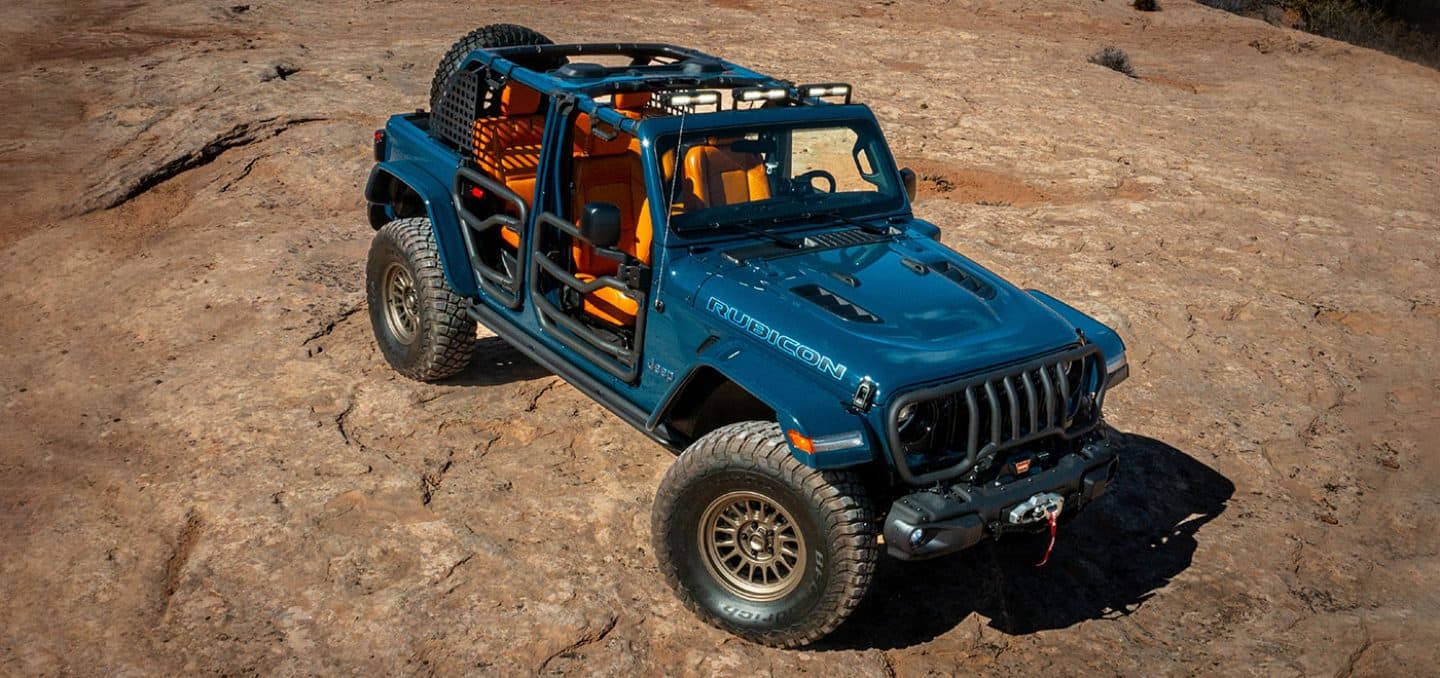A striking royal blue Jeep Rubicon is prominently featured in this horizontal photograph. The vehicle boasts a rugged and adventurous aesthetic, highlighted by its soft-top removed to reveal a vibrant orange leather interior. Its large tires underscore its off-road readiness, with a spare tire visibly mounted on the back. The name "Rubicon" is emblazoned in white lettering along the side of the Jeep, adding a touch of distinction. The front of the vehicle is marked by a black grille, which appears to be made from a durable plastic material. This robust Jeep is captured on a dirt road, emphasizing its capability for rugged terrains and outdoor exploration.